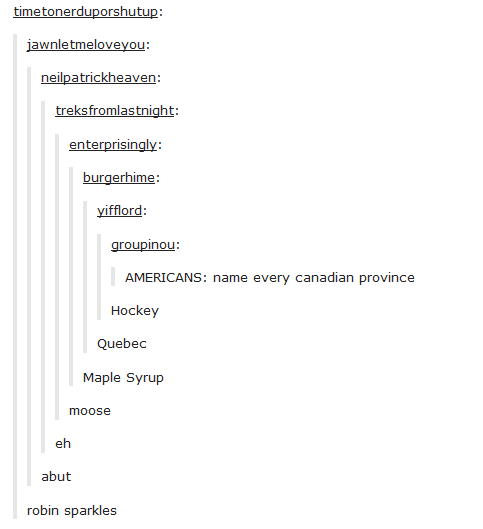The image depicts a chaotic yet symmetrical discussion thread from an online forum. The thread features numerous usernames like "Time," "Toner," "Doop," "Poor," "Shut Up," "Neil Patrick Heaven," and "Enterprisingly," all contributing to the conversation. In the center of the screen, a prompt reads, "Americans, name every Canadian province." Around this prompt, various users have posted humorous and arbitrary responses such as "Hockey," "Quebec," "Maple Syrup," "Moose," "Eh," "Abut," and "Robin Sparkles." The presentation of the thread, though visually symmetrical, makes it challenging to follow the conversation, adding to the comedic confusion.